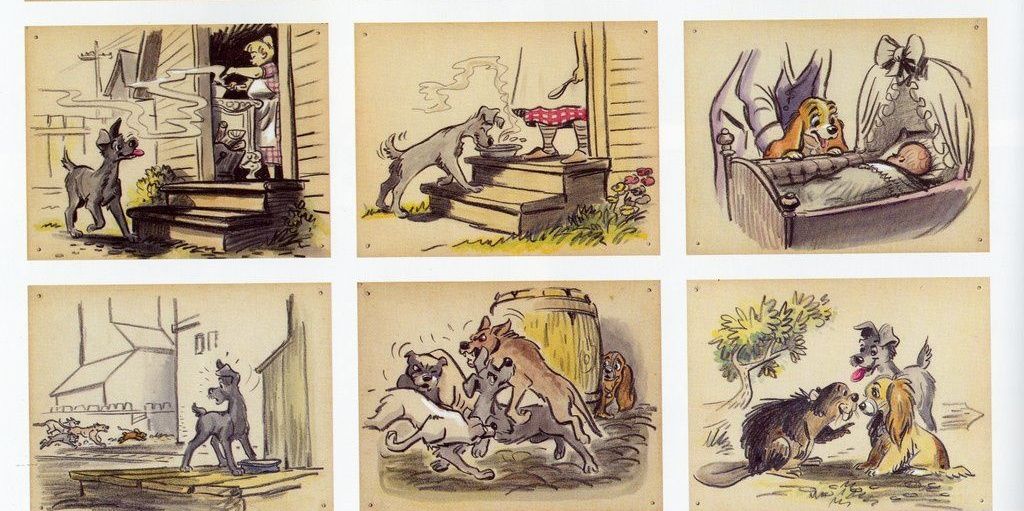This image is a detailed grid of storyboard illustrations reminiscent of the Disney movie, *The Lady and the Tramp*. The storyboard is set in a sepia-toned background, giving it an old comic strip feel. Arranged in two rows of three illustrations each, the scenes unfold as follows:

1. In the first image, a grey dog is seen walking past a woman's front door while she cooks inside. The enticing aroma wafts out to the dog.
2. The second image shows the woman standing at the doorway, placing a silver tray of food on the step. The grey dog eagerly starts eating from the dish.
3. The third image features the Tramp, a female dog, looking into a bassinet with a newborn baby inside. A woman stands behind the dog.
4. Moving to the bottom row, the grey dog is again seen eating on the steps but then turns his attention toward a pack of dogs running in the distance.
5. The fifth illustration depicts the grey dog in a struggle, potentially fighting off these stray dogs while the female dog hides behind a nearby barrel, watching the confrontation.
6. The final image in the bottom right-hand corner shows the grey dog and the little brown female dog, now conversing with a little brown beaver, emphasizing a collaborative dynamic as they come together.

This sequence portrays themes of companionship and protection, with the grey dog protecting others and the distinct contrast between scenes of domestic tranquility and street survival.